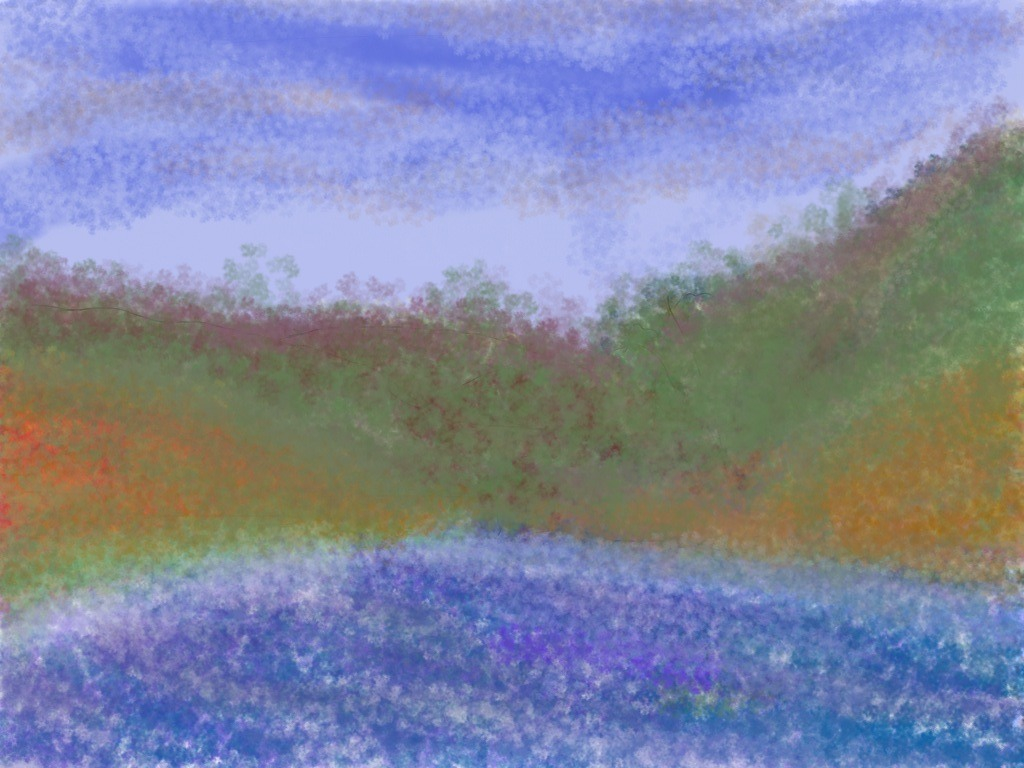A vibrant painting with a distinctive blotchy, sponge-painted texture captures the eye. The composition begins with a serene waterway at the bottom, possibly a lake or pond, characterized by deep blues and tranquil ripples. Above the water, a sandy shoreline emerges, transitioning gradually from taupe at the water's edge to earthy greens as it ascends. The upper edge of the ground is tinged with a subtle purple hue, adding depth and contrast. The sky above is an ethereal blend of white and soft blue, evoking a peaceful, possibly early morning or late afternoon, setting. The artist's use of color and texture creates a dynamic and immersive landscape scene.